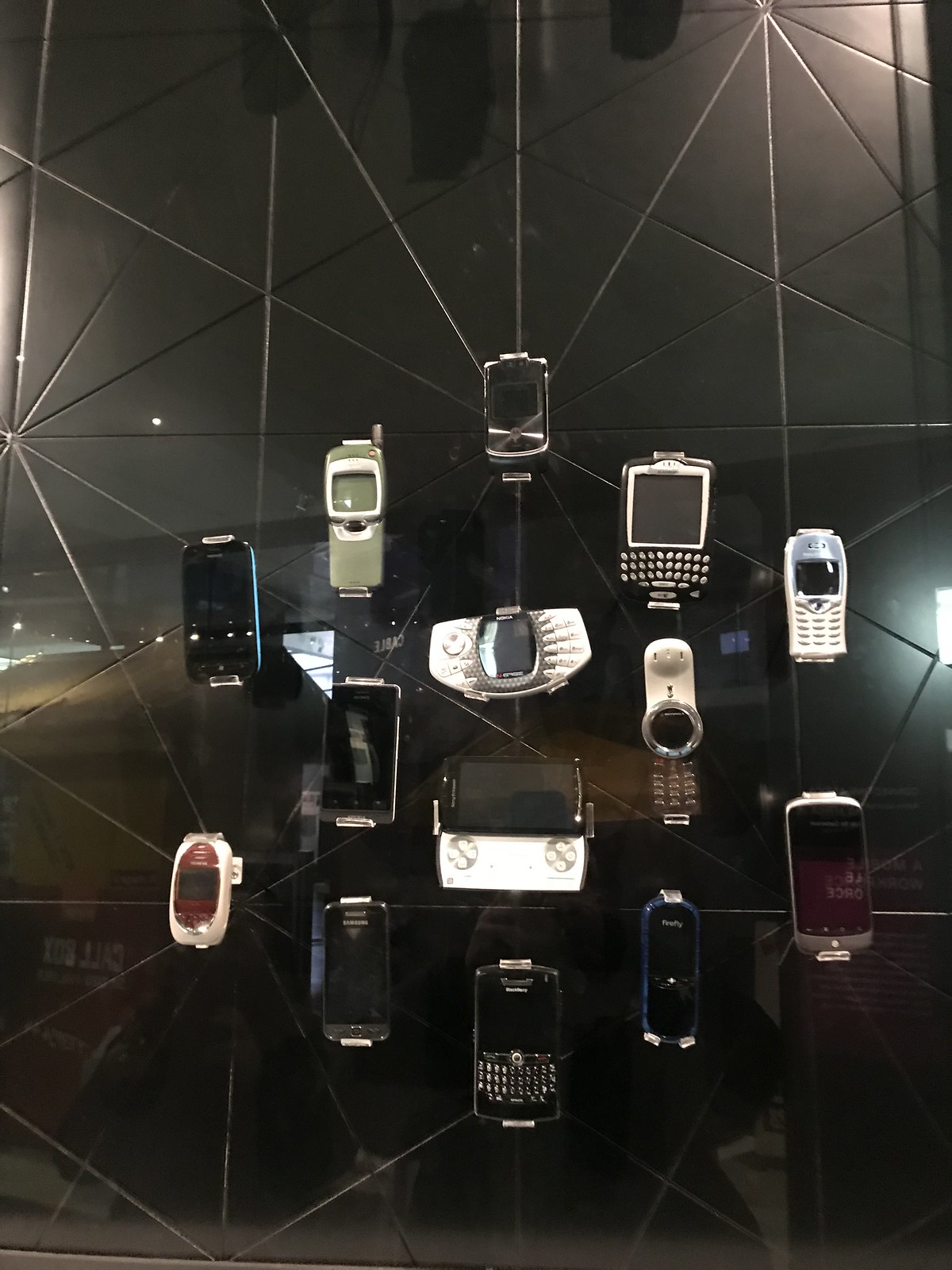This detailed photo showcases an array of vintage cell phones, primarily from the early 2000s. The collection features around 10 devices, carefully arranged on a cracked, reflective glass surface. Among the phones, there are various models such as Blackberries, flip phones, and slide phones, including some with slide-out keyboards and others with keyboards integrated onto the face. Notably, there's a black Blackberry, a Samsung that resembles modern designs, and a Motorola flip phone. The phones come in a variety of colors, including black, white, silver, purple, orange, and pink. Each phone is placed on a small stand for display, accentuating their unique design characteristics against a stark black background.